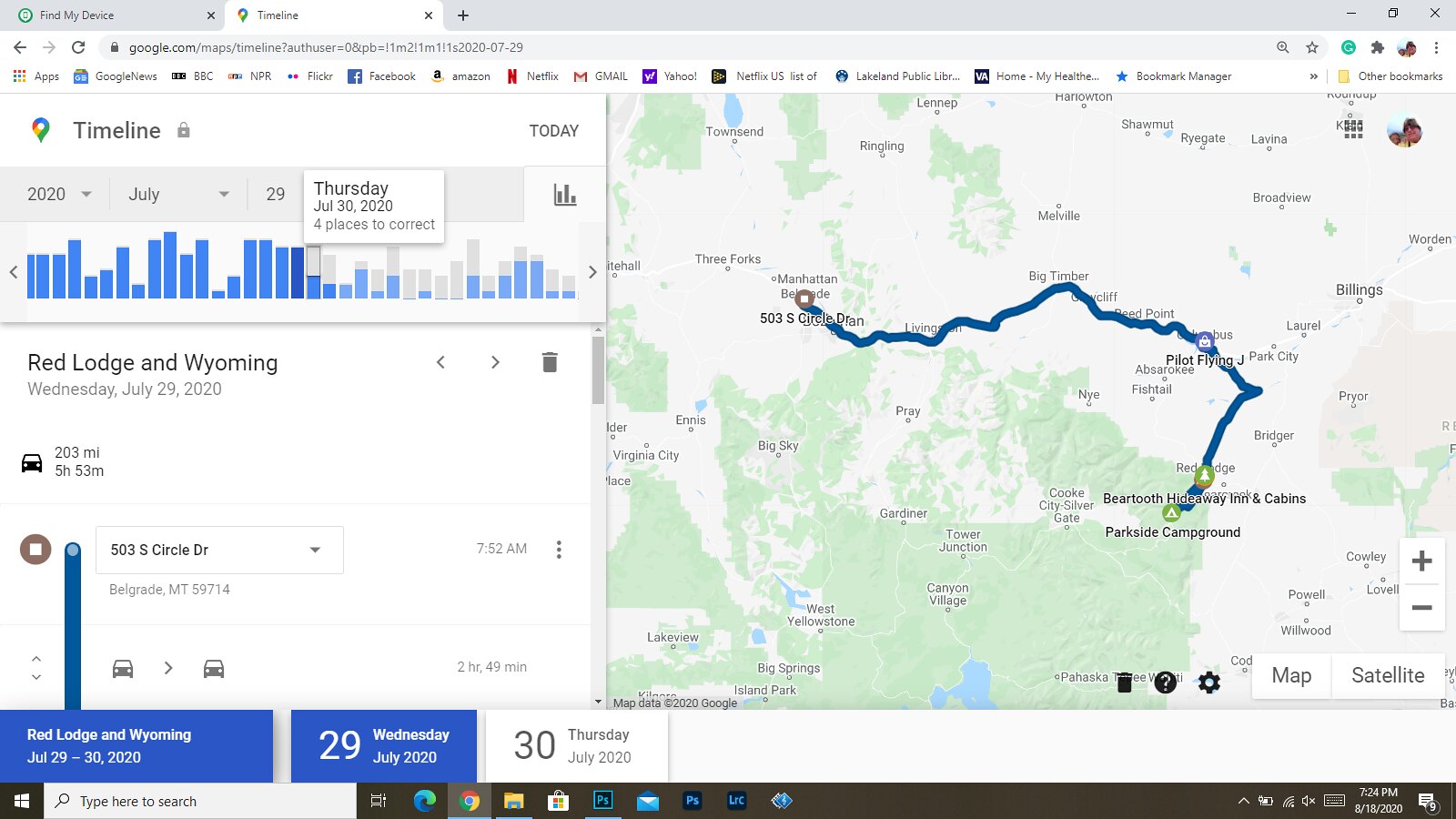This screenshot captures a detailed window of a Windows 10 desktop, prominently featuring the taskbar along the bottom edge with various open program icons and system status indicators like the clock and network. The desktop displays two active browser tabs: one titled "Find My Device" and another, currently visible, showcasing a detailed Google Maps timeline.

The visible tab details a journey plotted out on July 29, 2020, starting from Red Lodge, Wyoming, and ending in Belgrade, Montana. The trip spans a distance of 203 miles and lasted 5 hours and 53 minutes. The left pane of the browser tab provides this textual information, including a specific address: 503 South Circle Drive, Belgrade, MT 59714. Additionally, the date and day anomalies are noted at the bottom of the tab, showing Wednesday, July 29, 2020, while simultaneously stating the "33rd day July 2020."

On the right side of the browser tab, the map visualizes the journey, with a line marking the route between the starting and ending points. The browser interface also includes navigational buttons and several shortcut icons to popular websites such as Facebook, Amazon, Netflix, Gmail, and Yahoo. The image is a comprehensive illustration of a digital journey log within a typical user interface of a Windows 10 environment.